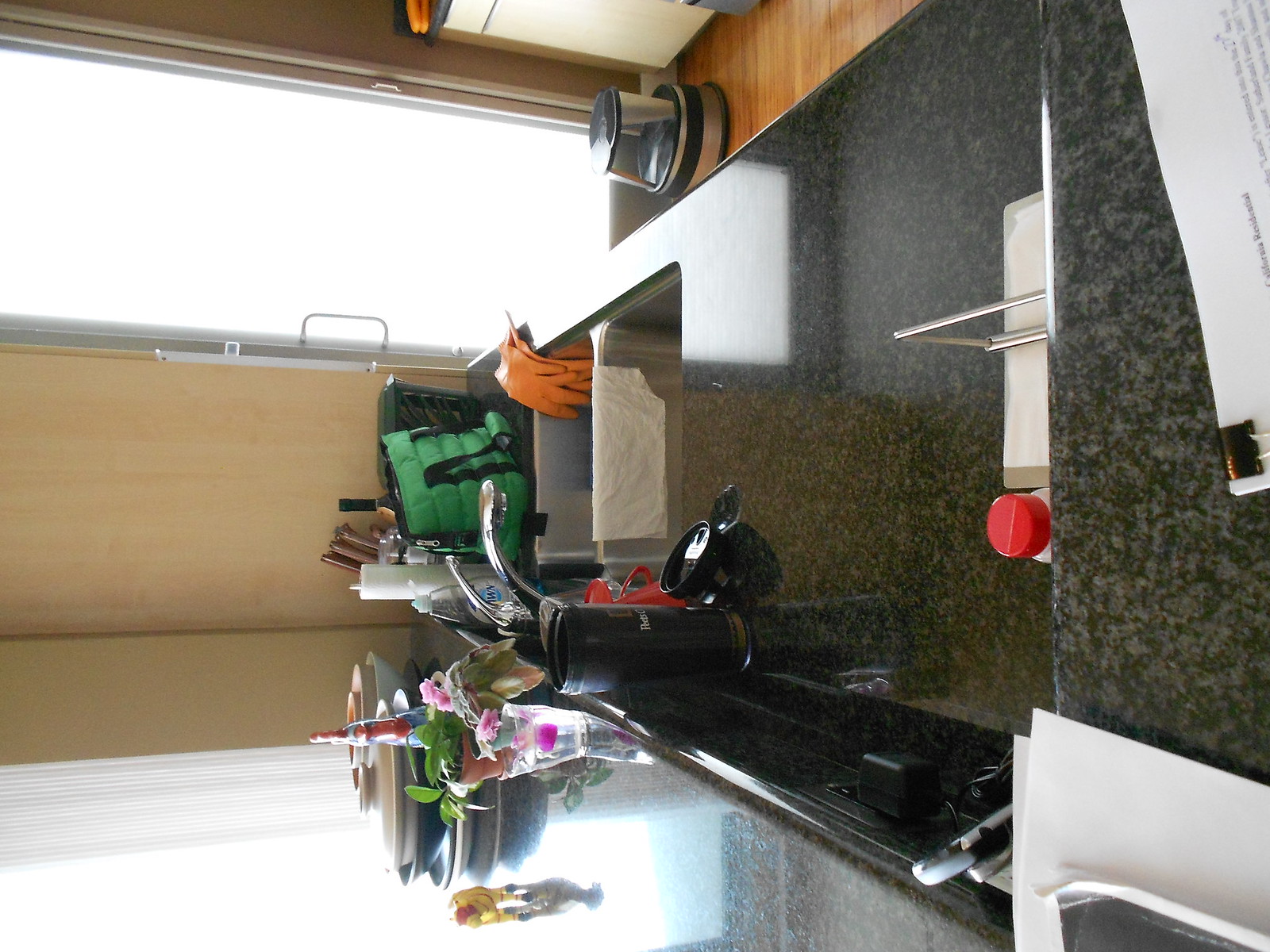An indoor color photograph showcases a unique angled view of a kitchen countertop. Positioned centrally, the countertop extends from the right edge of the frame into the background, ending slightly left of center. It features two stainless steel sink tubs, with a pair of orange gloves draped into the tub positioned further into the background. Adjacent to the end of the countertop, a green bag sits with an unidentified object protruding leftward from it, and a tan wall spans the background from the counter to the left edge of the frame. 

In the lower region of the image, a window is visible with a windowsill above it, supporting an assortment of pots and dishes. A small glass centerpiece, possibly a flower ornament, is also present. The area just right of center in the upper portion of the frame reveals a hardwood floor and a circular metal step stool. From left of center to the left edge, a vertical patio door allows white light to flood into the scene. In the upper right corner, a piece of paper clipped with a black metal clip intrudes slightly into the frame.